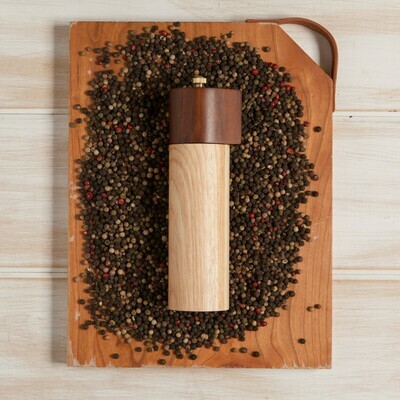The image features a richly detailed photograph of a two-tone wooden pepper grinder lying on a well-worn, rectangular cutting board with a distinctive top right corner cut-off at an angle. The pepper grinder itself has a cylindrical handle made of light beige wood, juxtaposed with a darker, rich cherry wood top that appears to be spinable. Surrounding the pepper grinder are an assortment of peppercorns in various colors including black, gray, red, yellow, beige, and green. The cutting board, aged and worn at the edges, sits on a light wooden surface that resembles a picnic table with a beige panel background. The entire composition is a nearly square vertical rectangle, with the peppercorns and grinder centrally arranged, giving the scene an indoor, tabletop setting with a rustic, culinary atmosphere.